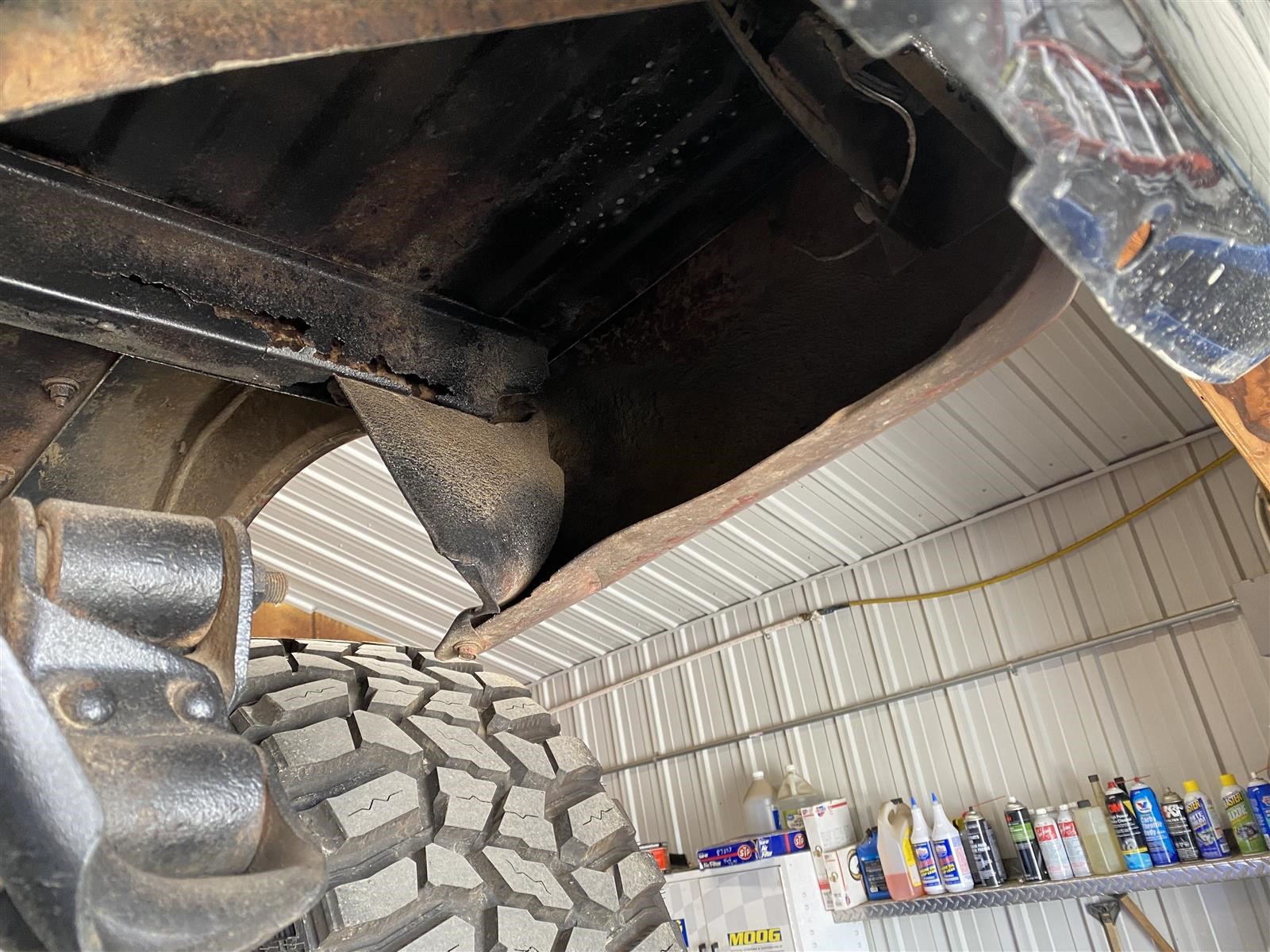In the image, we see an oddly shaped room that appears to be part of a vehicle's inside, likely a wheel well. To the bottom right, there is a grey shelving unit storing various automotive products. Notably, the shelf holds brake cleaner cans and a Seafoam bottle in the middle, which has a red banner with white edging on the outside and top. Adjacent to the Seafoam bottle, there is a black spray can on each side, and another clear plastic bottle with a mysterious brown substance.

The back wall and ceiling of the room are constructed of off-white metal panels featuring noticeable ridges. On the left side of the image, the grey tread of a tire is visible, hinting that the room is within a vehicle's wheel well. Below the tire, there is dark grey metal and what appears to be the rusted black body of the vehicle.

Above the shelving unit, there are white and yellow wires running across the ceiling, alongside a grey metal pipeline. To the left of the shelving unit is a white box marked "Moog" in yellow letters outlined with grey. Positioned on top of this box is a blue box, adding to the array of automotive supplies in the scene.